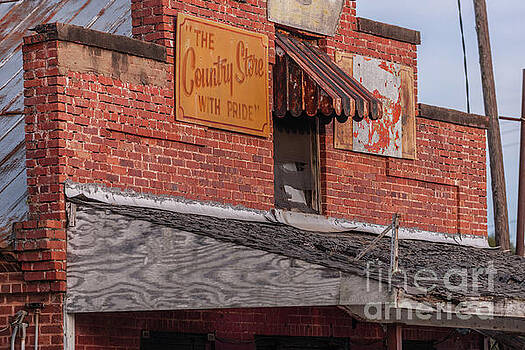The image captures the weathered façade of an old, possibly abandoned red brick building. Spanning horizontally, the photo focuses on the upper portion of what appears to be a historical storefront. A faded awning juts out above a central window flanked by two worn signs. The left sign, though aged, reads "The Country Store" in an old school style with fancy cursive and bold lettering, while the right sign is so deteriorated that its text is no longer legible. Below the signs, the building's exterior is covered by aged, gray, and severely weathered wooden planks, suggesting years of exposure to the elements. To the right of the brick structure, a telephone pole stands, adding to the rustic scenery. The angled view of the photo allows a glimpse of the side of the building, revealing another window on the left and some rusted tin roofing above the second story. The sky is a muted gray-blue, providing a somber backdrop to this relic of the past, with the bottom right corner of the image subtly marked with “Fine Art America” in transparent gray text.